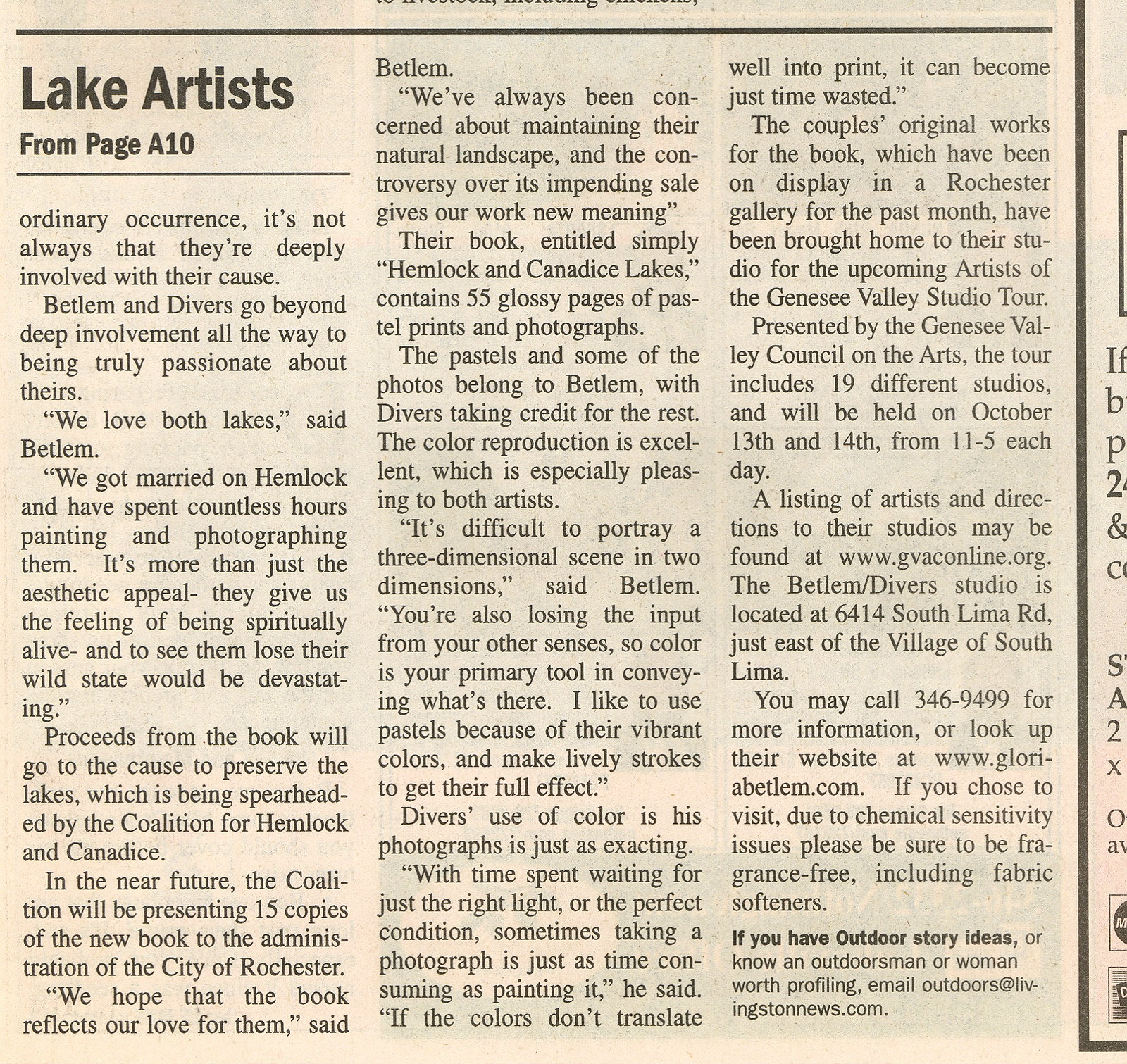This image is a newspaper clipping, titled "Lake Artists from page A10," set against a slightly aged, yellowish background. The headline introduces a detailed article about artists Betlam and Divers, who are profoundly passionate about preserving Hemlock and Canadas Lakes. Both artists, deeply connected to the lakes—they even got married on Hemlock—-have spent countless hours capturing the lakes' beauty through painting and photography. They express that their work is more than just appreciating the aesthetic; the lakes provide them with a sense of spiritual aliveness, and the possibility of losing their natural state is devastating. Their book, "Hemlock and Canadas Lakes," features 55 glossy pages of pastel prints and photographs, with proceeds aimed at the lakes' preservation, supported by the Coalition for Hemlock and Canadas. The article indicates future plans for the Coalition to present 15 copies of the book to the city administration of Rochester. Beyond detailing their artistic endeavors and conservation efforts, the clipping includes a call for outdoor story ideas and contact information for readers interested in contributing or learning more.